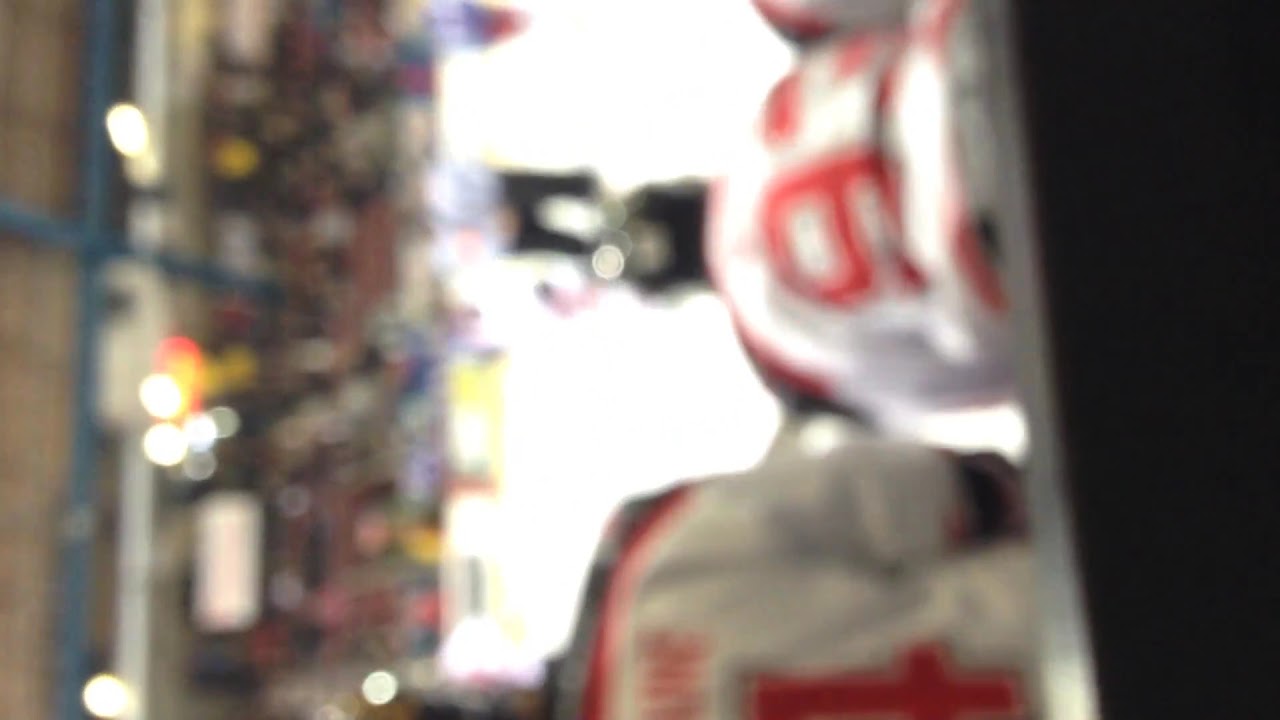This is a rectangular image rotated 90 degrees to the left, presenting a highly blurred and out-of-focus view of a sports arena, likely an ice hockey rink. In the scene, several individuals are discernible in red and white jerseys with numbers on their backs, including the number nine, seated on the boundary near their bags. They are positioned against a backdrop of an ongoing game, where blurred figures of players can be seen on the ice, along with someone standing in the middle, possibly holding a hockey stick. The stadium extends beyond the rink with indistinct, orange, yellow, and white lights scattered throughout, illuminating the setting. The stands are filled with an audience, though details are heavily obscured. Above, to the far left side of the rotated image, a brown ceiling with potential blue beams faintly emerges from the fuzzy depiction.